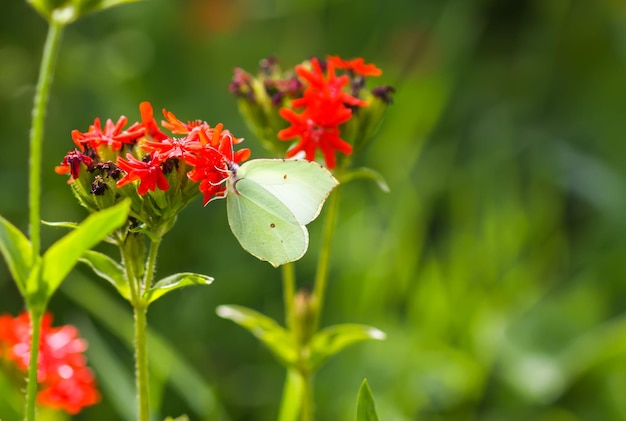The image captures a close-up view of thin, hairy-stemmed plants topped with bright red flowers. Perched on one of these blossoms is a predominantly off-white butterfly, notable for its long antennae and wings slightly spread away from its body. The butterfly appears to be sipping nectar from the red flower, which also has hints of purple in its petals. The insect’s wings display a slight greenish hue and are accented with small brown dots. In the blurred, green background, more red flowers can be observed, but this particular bloom, situated to the left, is the only one with a butterfly. The detailed, focused foreground stands out sharply against the soft, leafy backdrop, illuminating the intricate features of the scene.